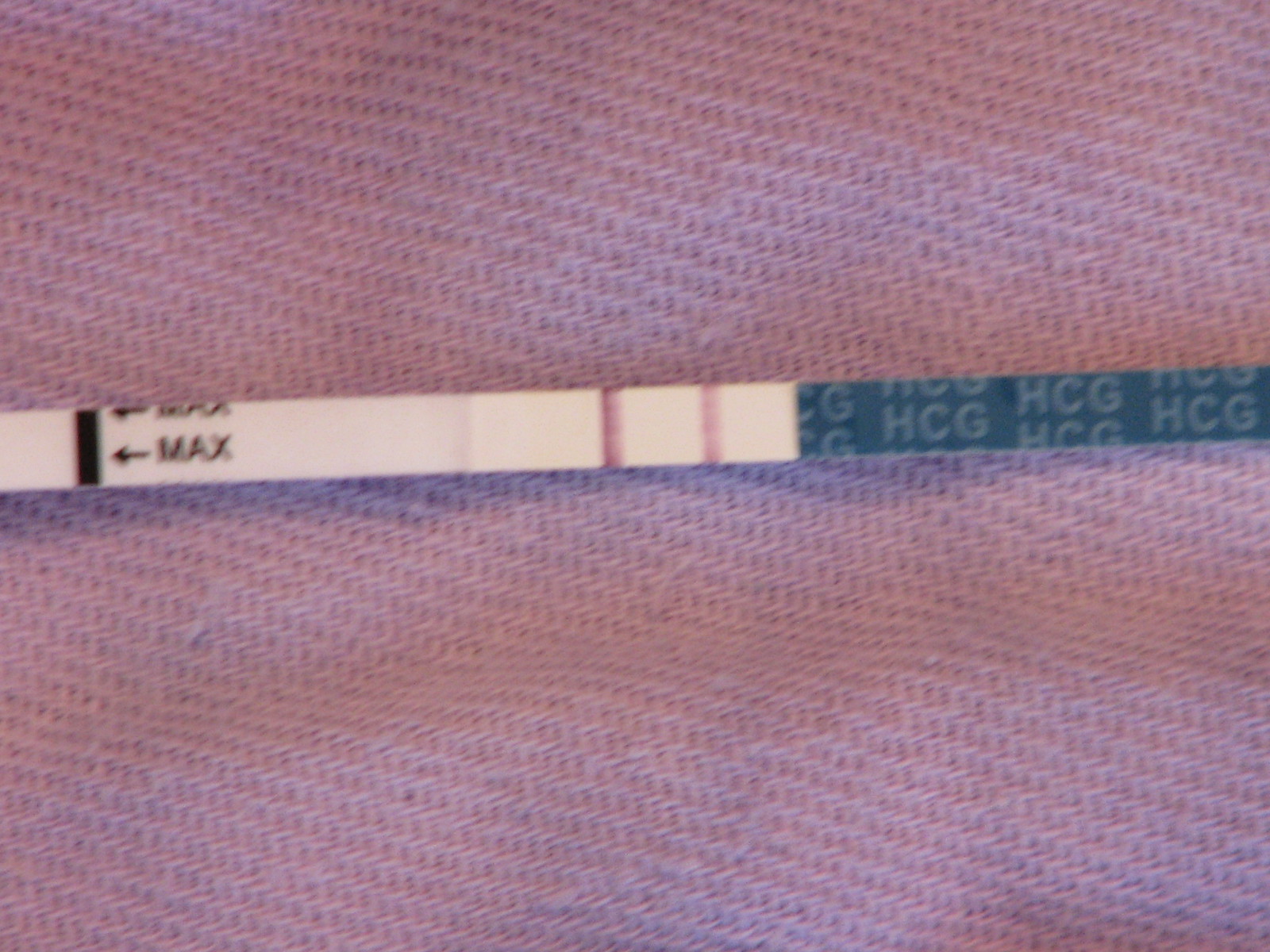The image showcases a close-up view of a slender test strip, positioned horizontally against a piece of burgundy cloth with a rough texture, reminiscent of a loose-weave washcloth. The left side of the test strip features the word "Max," although it appears blurry. On the right, the strip is labeled "HCG" multiple times in a repeating pattern. Between these labels, the test strip displays two lines in the middle, with the upper line being noticeably darker than the lower one. The strip itself is flat, approximately one centimeter in width, and stretches out of the frame, so its full length is not visible. The detailed presentation, hinting at its possible use as a dipstick or pregnancy test, emphasizes the importance of precision and context in interpreting the strip's results.